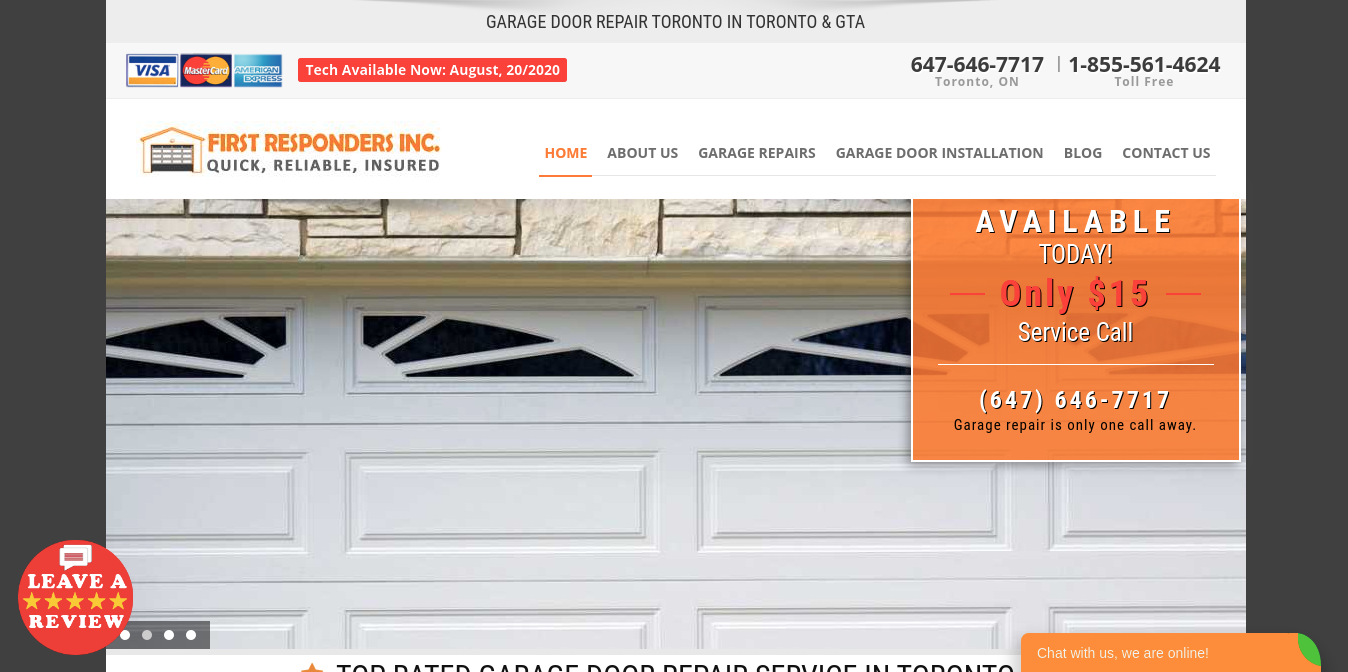This image displays a detailed view of a webpage belonging to a garage door repair service based in Toronto, known as "Garage Door Repair Toronto, in Toronto and GTA". At the top of the page, several credit card icons are visible for Visa, MasterCard, and American Express, indicating the accepted payment methods. A prominent button reading "Tech Available Now, August 20, 2020" is located below these icons. To the right, the contact details are displayed: a local phone number, 647-646-7717 for Toronto, Ontario, and a toll-free number, 1-855-561-4624.

The webpage is hosted by "First Responders, Inc.", and their tagline is "Quick, Reliable, Insured". The navigation menu includes tabs for Home, About Us, Garage Repairs, Garage Door Installation, Blog, and Contact Us, with the Home tab currently active. 

Further down the page, an image of a white garage door is shown. In the lower left, there is a prompt for users to "Leave a Review". On the right side, a promotional message reads "Available Today, Only $15 Service Call", accompanied by the phone number 647-646-7717 again. Below this, a small sign on the garage door emphasizes, "Garage Repair is only one call away".

Overall, this webpage portrays a garage repair service, highlighting their reliability and accessibility for customers needing urgent garage door repairs.